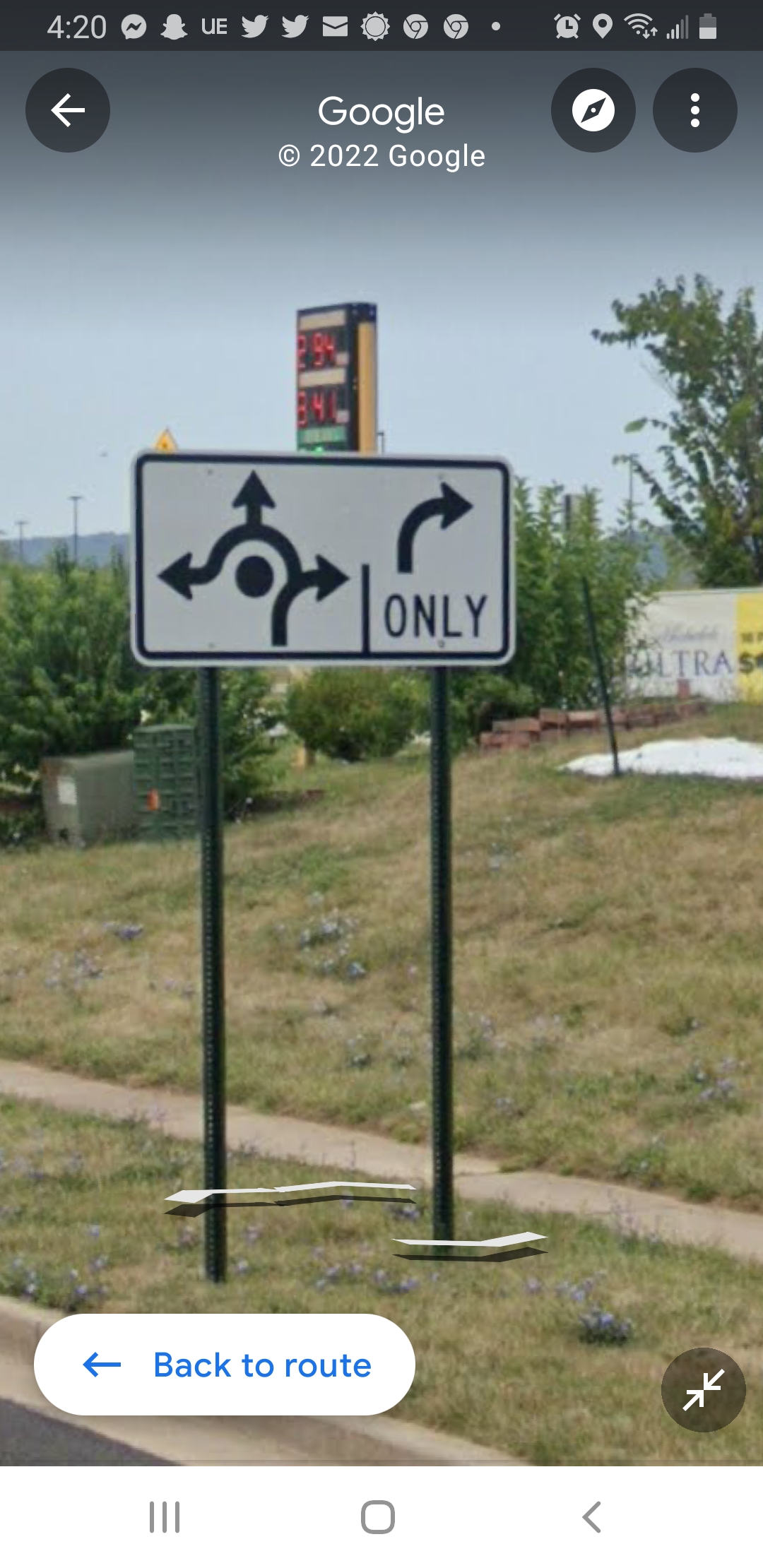The screenshot, captured from a phone displaying the Google Maps UI, shows the time (4:20) along with various app icons like Messenger, Snapchat, Twitter, and Gmail at the top. The screen displays a navigation view with a “Back to route” option at the bottom. The focus is on a road sign standing on two poles amidst grassy surroundings. The white sign, indicating a roundabout ahead and a right turn only, features a filled circle and a half-circle with three arrows pointing in different directions. In the background, there is a gas station with a neon red sign displaying fuel prices—$2.94 and $3.41—alongside some electrical boxes, trees, and a sidewalk.